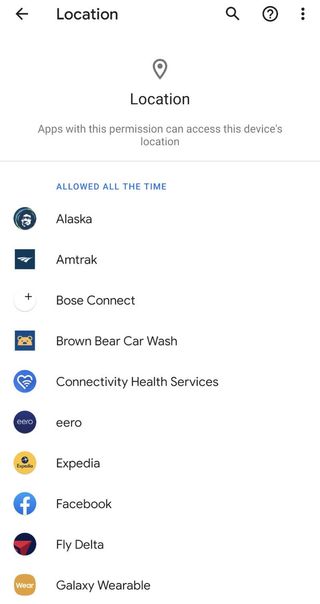The image is a screenshot taken from a mobile phone, displaying a settings page with the theme focused on "Location" permissions. The background of the page is white. At the top-center of the screen, the word "Location" is written prominently in bold black text. To the left of the title, there is a back-arrow icon, while to the right, there are two more icons—a magnifying glass with a question mark inside and a vertical ellipsis (three vertical dots).

Beneath the header, there is a small pin icon followed by the word "Location" written again. Below this, a description states: "Apps with this permission can access the device location." A thin gray line separates this section from the subsequent content.

Following the gray divider, there's a section titled "Allowed all the time" written in blue text. This section lists various apps that have been granted continuous location access. The apps mentioned include:

- Alaska
- Amtrak
- Bose Connect
- Bear Brown Car Wash
- Connectivity Health Services
- Aero
- Expedia
- Facebook
- Fly Delta
- Galaxy Wearable

Each app name is accompanied by its corresponding icon to the left. Notably, the icon for Bose Connect is a simple white circle with a plus sign inside, the icon for Bear Brown features an image of a bear, and the Facebook icon is represented by a lowercase 'f'.

This detailed layout captures the structure and appearance of the settings page regarding location permissions on the device.